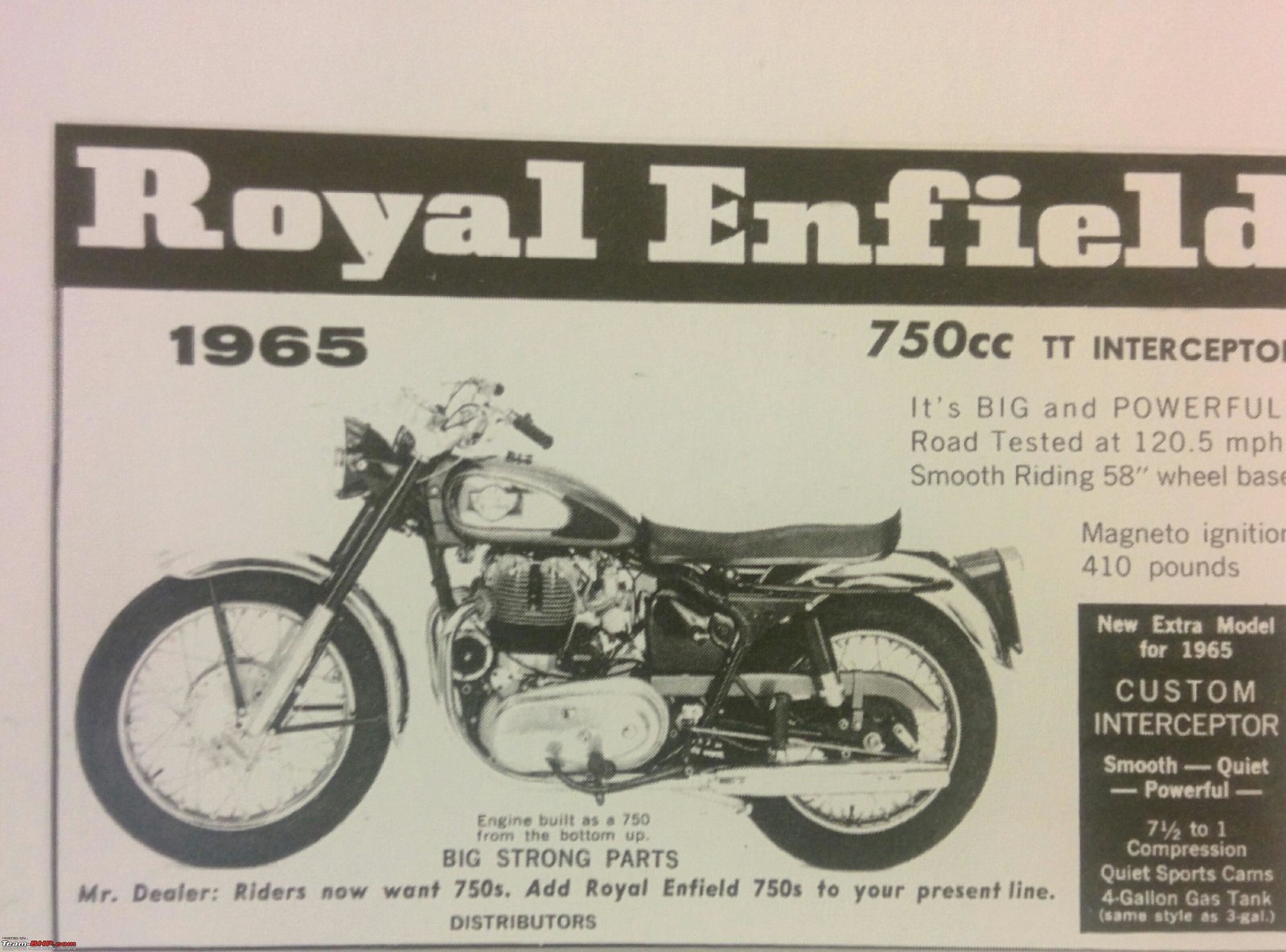The image is a zoomed-in, black and white advertisement from an old magazine, featuring a side profile photograph of a Royal Enfield motorcycle, specifically the 1965 750cc TT Interceptor. The motorcycle's front wheel points left while the back wheel points right. The ad has a stark black border at the top with the bold text "Royal Enfield" prominently displayed. Below this, in smaller black font on a white background, it reads "1965, 750cc, TT Interceptor."

The bike, showcased in gleaming chrome with detailed fenders, looks brand new despite the vintage feel of the ad. To the right of the image, there are descriptive details emphasizing the bike's features: "Big and powerful," "road tested at 120.5 miles per hour," "smooth riding, 58-inch wheelbase," "Magneto ignition," and weighing "410 pounds." It mentions the "new Essex model for 1965, custom Interceptor," with specifics such as "7.5 to 1 compression," "quiet sports cams," and a "4-gallon gas tank, same style as 3-gallon."

Below the motorcycle, additional text highlights the engine's robust design: "Engine built as 750 from bottom up, big strong parts." The ad concludes with a call to action for dealers: "Mr. Dealer, riders now want 750s, add Royal Enfield 750s to your present line."